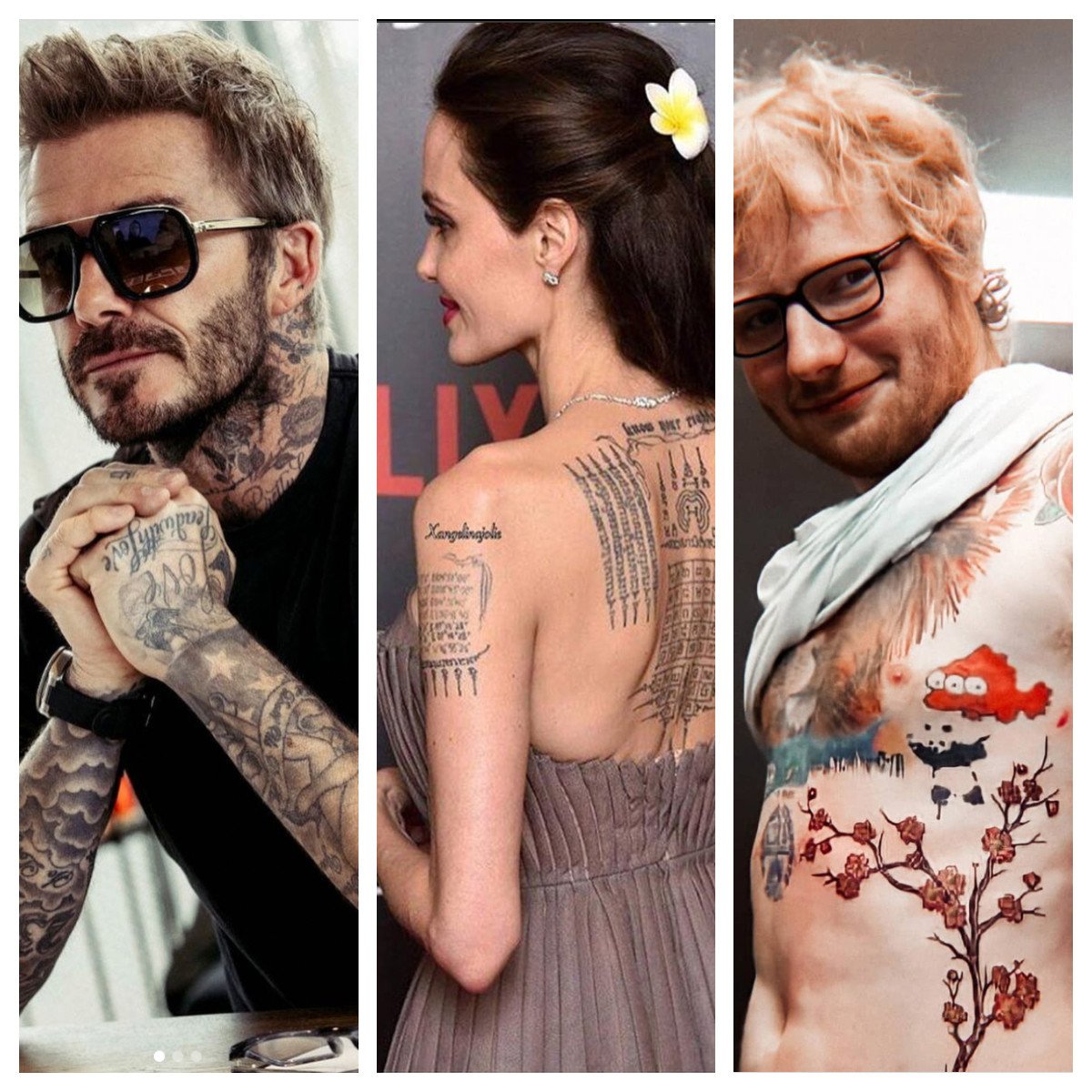The image comprises three rectangular photos aligned in a row, each separated by a white line. 

The first photo features David Beckham, a white male with light brown hair and a goatee. He is wearing sunglasses, a black t-shirt, and a black wristwatch. His hands are clasped in front of him, revealing tattoos that adorn his neck, arms, and hands.

The second photo captures Angelina Jolie in profile, her dark brown hair adorned with a Hawaiian-style flower, possibly a magnolia. She is wearing silver earrings, a silver necklace, and a sleeveless grey dress. Jolie's left arm showcases intricate tattoos, and her back is also tattooed with various designs.

The third photo shows musician Ed Sheeran with ginger red hair and regular glasses. He is smiling and has some facial hair. Ed's shirt is pulled up around his neck, revealing tattoos on his chest and side. Among the visible tattoos are a three-eyed fish, cherry blossoms, and other less discernible images.